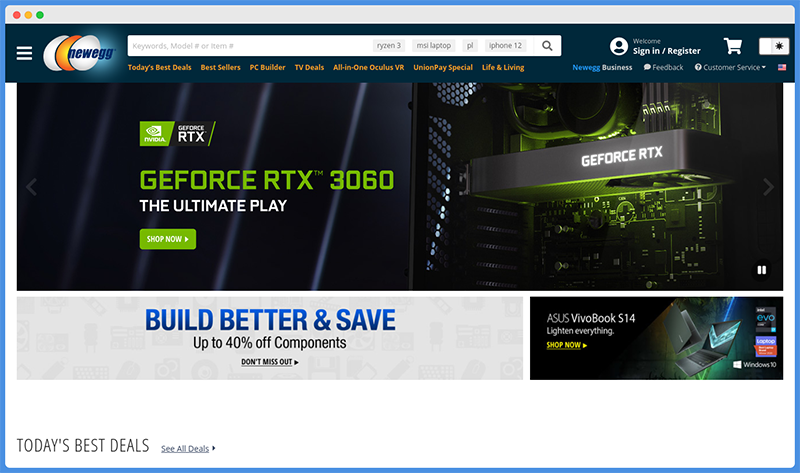The new Newegg website features a sleek and modern design. In the top left corner, there are three stylized eggs with dark blue outlines: the two outer eggs are white, while the middle egg is orange with a glowing yellow dot inside. The brand name "Newegg" is prominently displayed in a blocky, italicized dark blue font next to these eggs. 

To the right of this logo is a long white search bar, making it easy for users to find what they need. Adjacent to the search bar, there is a user icon followed by the text "Sign In / Register" in white lettering. Additionally, there is an icon of a white shopping cart to facilitate smooth shopping experiences.

Below this header, a menu bar with various options is displayed in small orange font. The categories listed include "Today's Best Deals," "Best Sellers," "PC Builder," "TV Deals," "All-in-One Oculus VR," "UnionPay Special," and "Life and Living." Towards the far right of this menu, "Newegg Business" is highlighted in blue, accompanied by a white comment icon labeled "Feedback," and a white-filled circle with a question mark indicating "Customer Service," which features a dropdown menu. Lastly, there is a small square icon of the American flag.

The main banner on the website showcases a slanted lime-green square logo with white iconography and text. Next to the logo, the letters "RTX" are displayed in white digital font, followed by a green forward slash. Further down, the text "GeForce RTX™ 3060" is written, with "GeForce" fully capitalized and the entire text featuring a registered trademark symbol in the upper right corner. This banner clearly highlights the promotion of the Nvidia GeForce RTX 3060 graphics card.